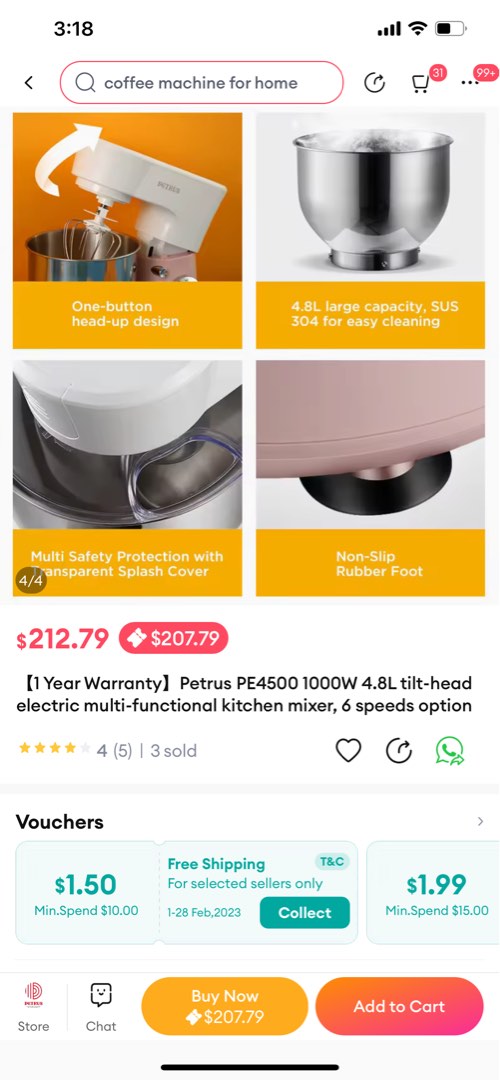The image depicts a mobile phone screen displaying a kitchen appliance shopping interface. At the top of the screen, the status bar shows the time "3:18" on the left, with icons for cell signal, Wi-Fi, and a half-full battery on the right. Directly below is a navigation bar with a back arrow and a search field containing the term "coffee machine for home." There is a shopping cart icon with "31" items and a three-dot menu with a red notification bubble indicating "99+."

Visible items include four product images with descriptions. The first product has a "one-button, head-up design." The second product features a "4.8L large capacity" with "SUS304 for easy cleaning." The third product, found on the lower left, offers "multi-safety protection" with a transparent splash cover, while the fourth product on the lower right has a "non-slip rubber foot." 

The price of one of the items is listed as "$212.79," struck through with a red circle indicating a discounted price of "$207.79." Details include a "one-year warranty," the model "Petrus PE4500," specifications of "1,000W, 4.8L," and "tilt head electric multifunction kitchen mixer," available with "six-speed options." The product boasts a four-star rating based on five reviews, with three units sold and a mention of a "$1.00 voucher" available.